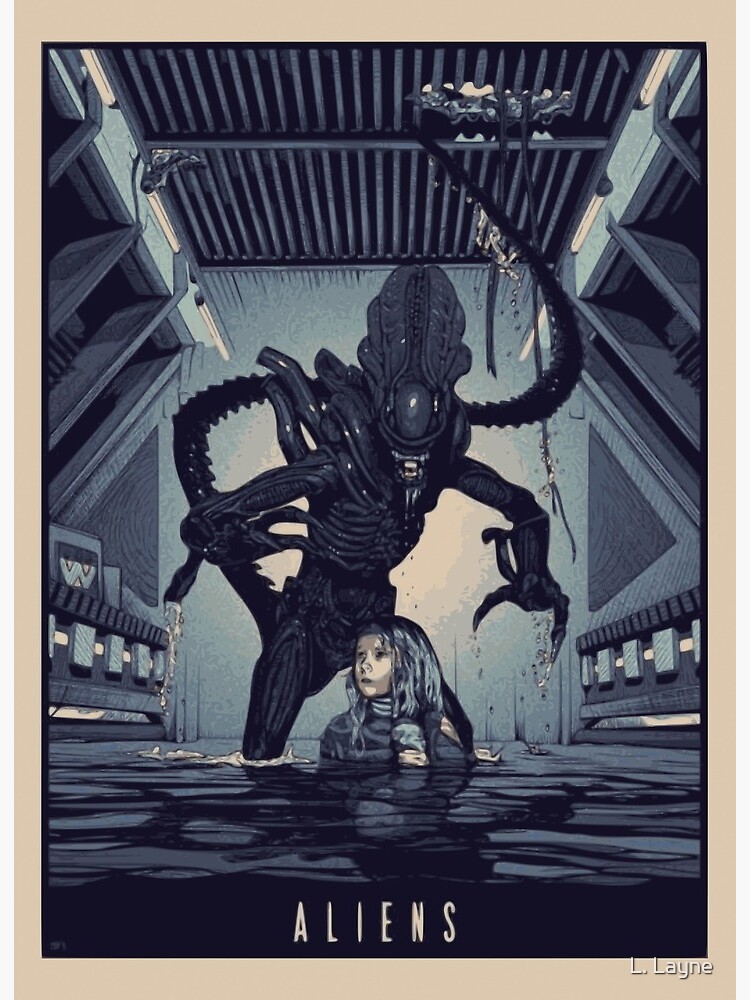This vertical rectangular movie poster for "Aliens" showcases a dramatic, stylized scene in a comic strip art style. The poster features a beige border and prominently displays the title "Aliens" at the bottom in bold white letters, with the text "L. L-A-Y-N-E" in the bottom right corner. The setting appears to be a dark, metallic indoor environment, likely a spaceship or sewer, with lighted panels and sewer grates visible above.

Central to the image is a little girl with shoulder-length dark hair, submerged in murky water up to her chest, exuding a sense of vulnerability and fear. The menacing alien, depicted as a monstrous creature constructed of metal, stands menacingly over her. The alien's terrifying features include multiple arms, some ending in sharp claws, and a gaping mouth filled with numerous teeth. Extending from its back is a long, tentacle-like appendage that arches upward and attaches to the ceiling through a hole. A tail and possible wing-like structures add to its nightmarish appearance. The scene is bathed in eerie lighting, with a faint glow emanating behind the alien, highlighting the tension-filled moment where it appears poised to grab the girl.